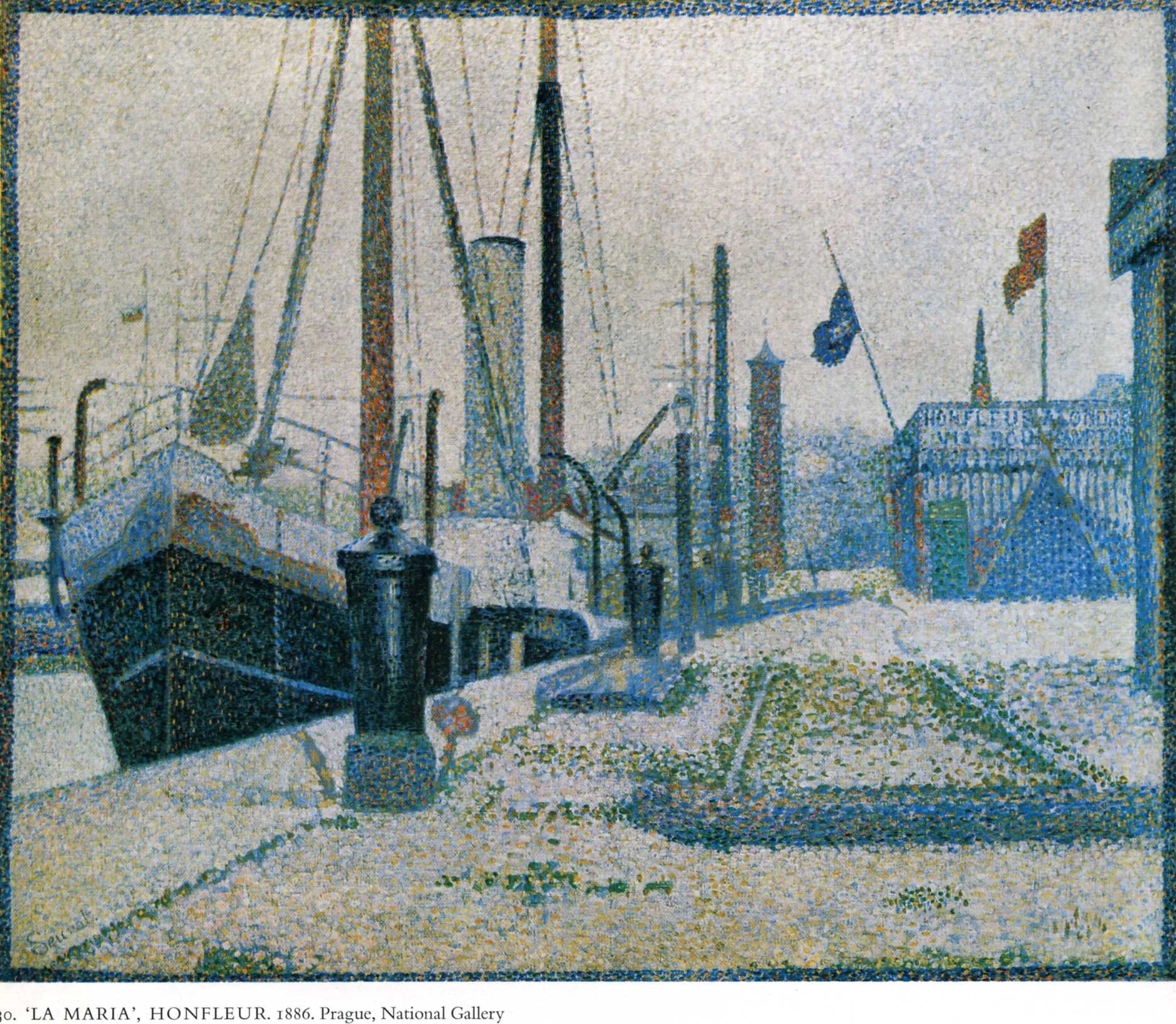This evocative painting, titled "La Maria" by the possibly French artist Honfleur, dates back to 1886 and is displayed in the Prague National Gallery. The artwork showcases an impressionistic or pointillistic style, characterized by dots and delicate paint strokes that conjure the image of a docked boat, emphasized in black and white hues. The boat, the central focus, bears a white upper section and is safeguarded by a silver metal fence running along its sides. The scene around the boat is adorned with vibrant accents; notable are the blue and rose-colored flags on the right, likely affixed to a nearby building or fenced structure. The setting is imbued with a subdued palette, featuring colors like grays, blues, greens, yellows, reds, and browns, enveloped in a somewhat dull, gray sky. The ground appears white, perhaps covered in snow, augmenting the serene atmosphere. Heavy black piers and tall ship masts reside in the background, with no visible human presence, directing all attention to the boat and its surroundings. The caption at the bottom reads "La Maria" with the artist's name and the exhibition details, grounding the historical context of this artwork in the Prague National Gallery.